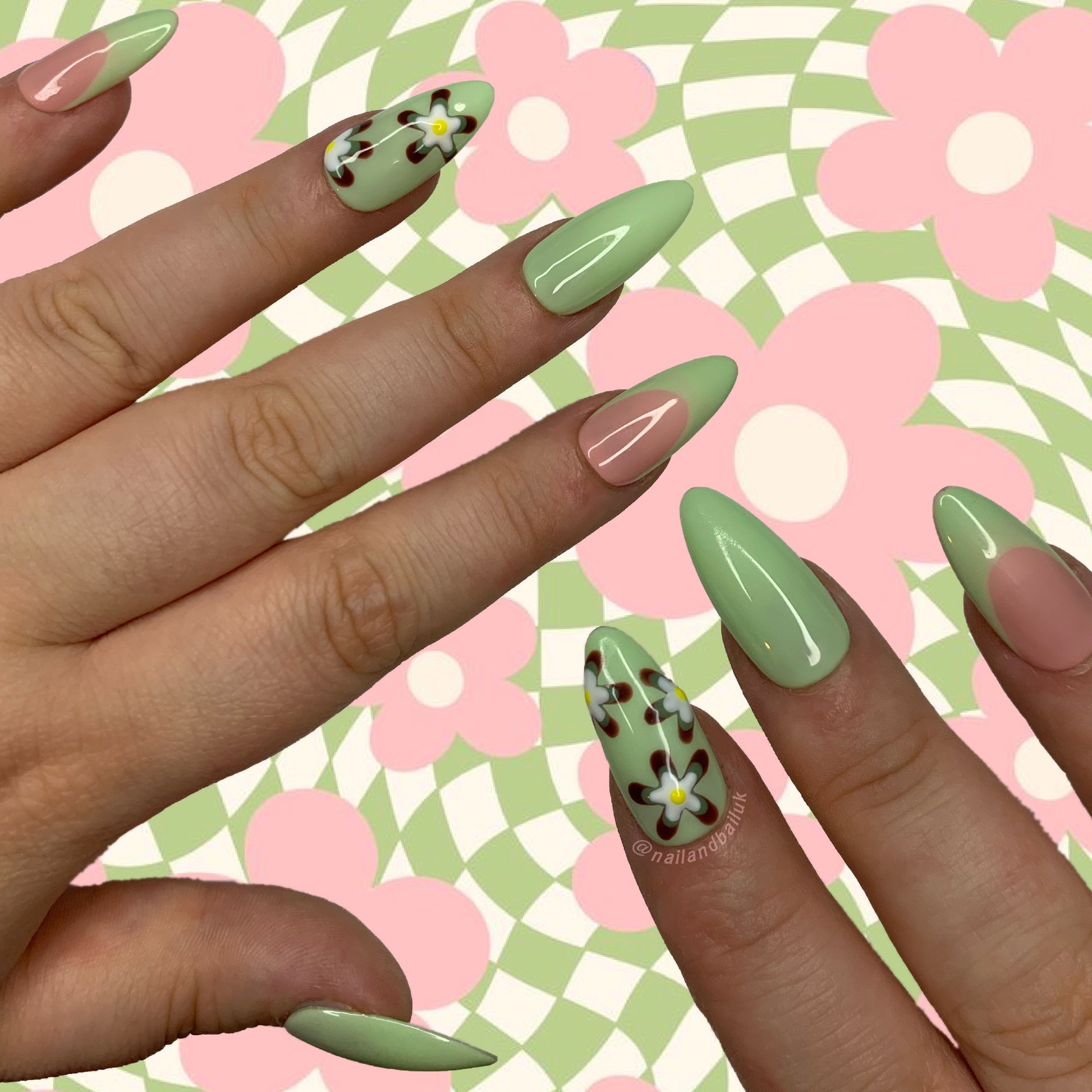This close-up photograph captures the ornate manicure of a woman's chubby hands, which appear slightly swollen. The nails are long and predominantly painted in a pea-green color that matches the green in the background. Each fingernail boasts a unique design: some nails feature pink shading combined with the green, while others display intricate black-edged white flower patterns with a yellow center. The background complements the manicure, showcasing a distorted, digital checkerboard pattern in green and creamy white, overlaid with pink flowers. The composition reveals two hands, one emerging from the left side and the other from the bottom right, exposing the tips of their fingers. The nails are shiny and well-coordinated with the backdrop, including a distinctive touch where one fingernail has “@NailAndBailUK” written around its base, highlighting a website.